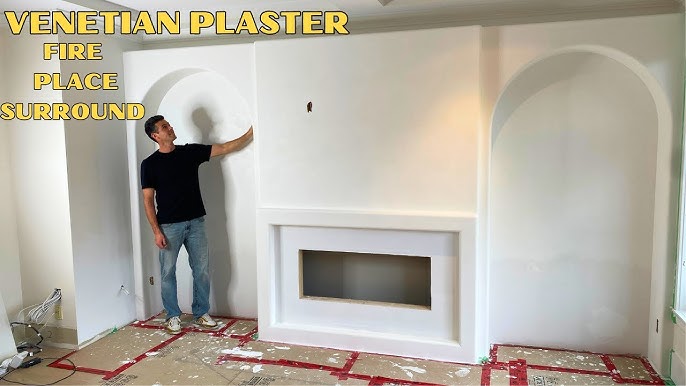The color photograph captures a living room undergoing renovations, featuring a predominantly white wall with a partially installed Venetian plaster fireplace surround, as indicated by the yellow text outlined in black in the upper left corner. The room is bare, with the floor covered in cardboard secured by red tape. Central to the image is a rectangular fireplace opening flanked by two shallow archways. Standing to the left of the fireplace opening is a man with dark brown hair, wearing a short-sleeved black t-shirt, blue jeans, and white-and-red trainers. His left hand is extended, touching the wall, and he's gazing upwards. Shadows cast on the wall behind him add depth to the scene. In the bottom left, an open outlet with visible wires hints at the ongoing electrical work, and the presence of an exterior window on the right side provides a glimpse of the outside.